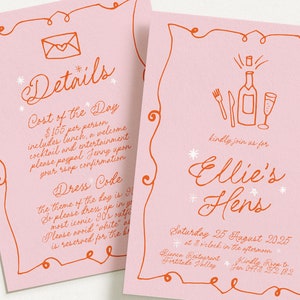This photograph showcases both the front and back of an invitation to a party titled "Ellie's Hens," scheduled for Saturday, August 25th, 2025, at 2:00 PM. The invitation consists of two pink cards with a detailed orange squiggly line border. The front card, positioned to the right, features an orange line drawing of an opened wine bottle in the center, flanked by a wine glass on the right and a fork and knife on the left. The text on this card, written in elegant cursive, reads: "Kindly join me for Ellie's Hens, Saturday, 25 August 2025." The back card, slightly covered by the front card on the bottom left corner, also has cursive writing in the same orange color and an illustration of an envelope sealed with a heart at the top. This card contains the heading "Details" and mentions the cost of $155 per person, which includes lunch, a welcome cocktail, and entertainment. It also refers to a PayPal account for confirmation and mentions a dress code with the theme, although much of this text is hard to discern due to its small size and cursive style.